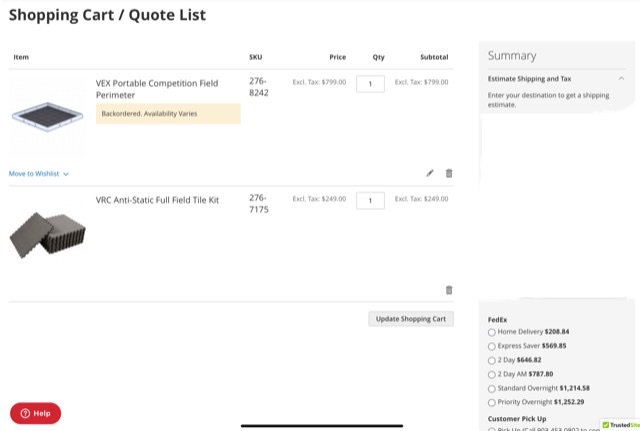The image displays a shopping cart interface dedicated to solar panel equipment or related items, set against a white background. In the upper-left corner, the header reads "Shopping Cart / Quote List." Below this, in bold black lettering, are columns labeled: Item, SKU, Price, Quantity, and Subtotal.

The first listed item is the "VEX Portable Competition Field Perimeter," accompanied by a small thumbnail image of the product on the left. Directly underneath this item name, an orange bar with black text states "Availability varies." To the right, the SKU number "2768242" is displayed, followed by the price "$799" (excluding tax) and a quantity of "1," resulting in a subtotal of "$799" (excluding tax). Below this, a blue hyperlink labeled "Move to wishlist" with a dropdown menu is positioned to the left, adjacent to icons for editing (pencil) and deleting (trash can).

The next item listed is the "VRC Antistatic Full Field Tile Kit," also accompanied by a corresponding product image on the left. The item's SKU, "276-7175," is shown to the right, followed by a price of "$249" (excluding tax) and a quantity of "1," leading to a subtotal of "$249" (excluding tax). Below this, a trash can icon is provided for deletion.

At the bottom of the cart, there is a button labeled "Update Shopping Cart." In the lower left, a red button with a question mark icon reads "Help." To the right of this button, a summary section includes various FedEx shipping options, detailing the different delivery methods available.